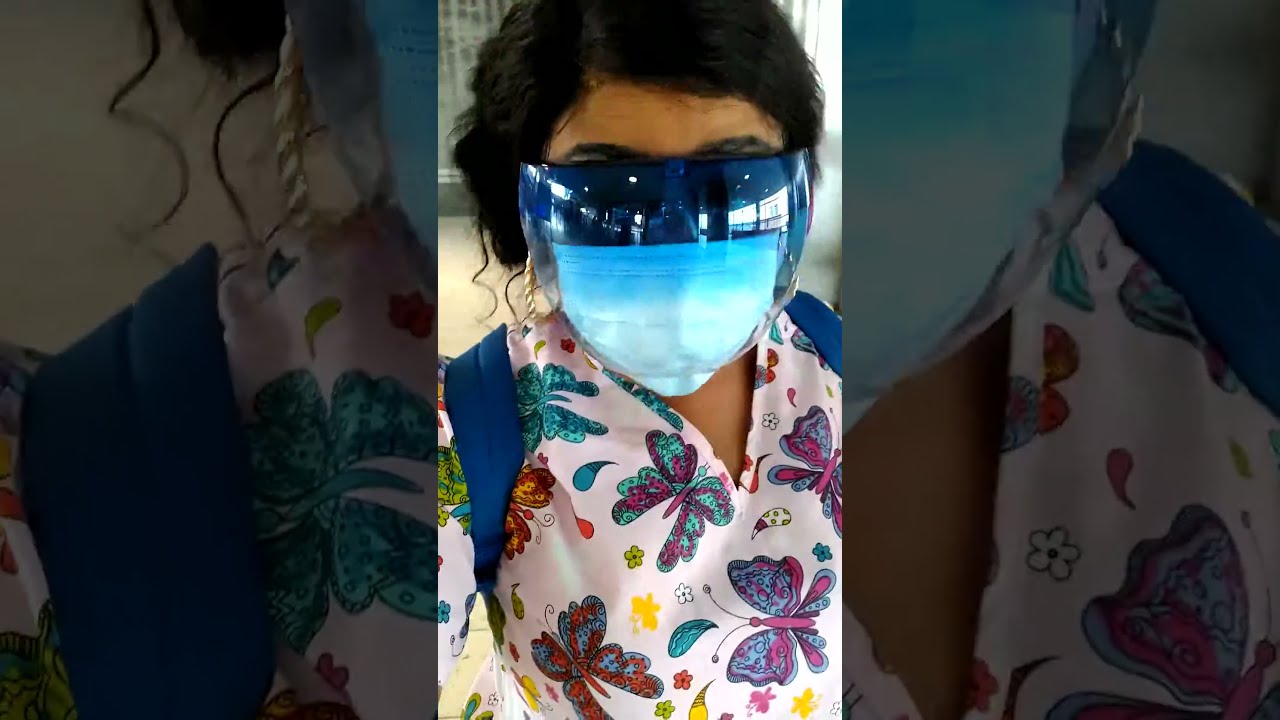The central image in the triptych displays a middle-aged woman of possible Hispanic or South Asian descent, with olive-brown skin and dark hair, donning a variety of safety gear. In the bright central photo, she wears dark blue, translucent safety goggles that provide a partial view of her eyes and catch reflections of window light. Additionally, she has a blue medical face mask, resembling those commonly used during the Covid-19 pandemic. Her outfit is a potentially medical scrub top adorned with an assortment of colorful butterflies in teal, purple, red, orange, and yellow, complemented by green and white floral patterns. Blue backpack straps cross her shoulders, suggesting she might be on her way to or from work. Gold, rope-design earrings peep out subtly from her dark hair.

The left section of the image is a close-up focusing on her right shoulder, showcasing a large teal butterfly from her attire, a segment of the blue backpack strap, her dark hair, and the distinctive gold earring, which resembles a piece of twisted rope. The right section provides another detailed fragment of the image, this time zooming in on the side of her face shield, part of her face mask, the backpack strap, and more of the butterfly-decorated scrub fabric, offering a more intimate look at the materials and patterns.

Set up like a landscape triptych, the darker side panels balance the brighter center image, where she seems to be walking inside a building, capturing the moment with a selfie from a slightly downward angle.